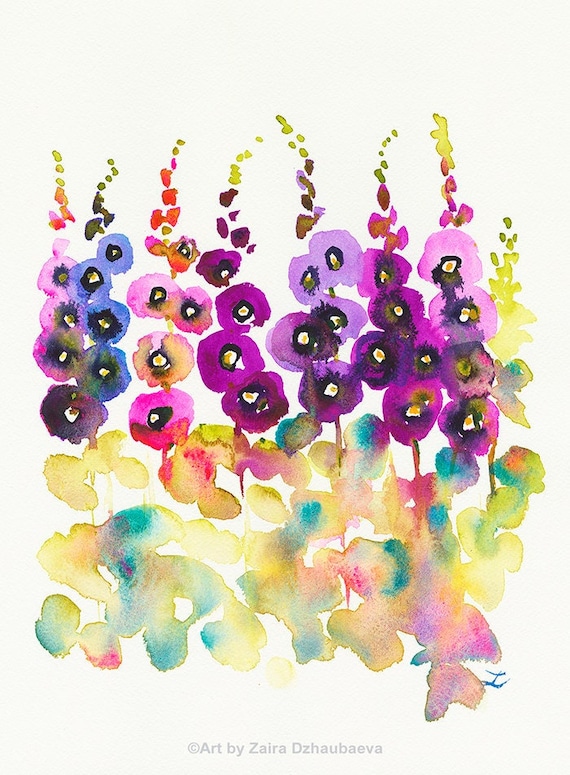This vertically aligned rectangular image showcases a watercolor painting on a beige page, embellished at the bottom with the inscription "© Art by Zahra Dzhubaeva" in gray print. The painting itself is an impressionistic, almost abstract depiction of flowers that resemble pansies. The lower half is dominated by large, light brown and yellow petals with hints of green and purple, possibly representing leaves. Extending from the middle to the upper part of the image, there are vividly colored, round-shaped flowers with varied hues. Each flower features an inner black circle with a white and yellow spot in its center, and an outer circle that ranges in color from purple and light purple to blue and pink. The flowers are arranged in a vine-like pattern with brighter colors ascending and more faded shades descending, connected by rainbow-colored stems and leaves, creating a harmonious and vibrant composition.